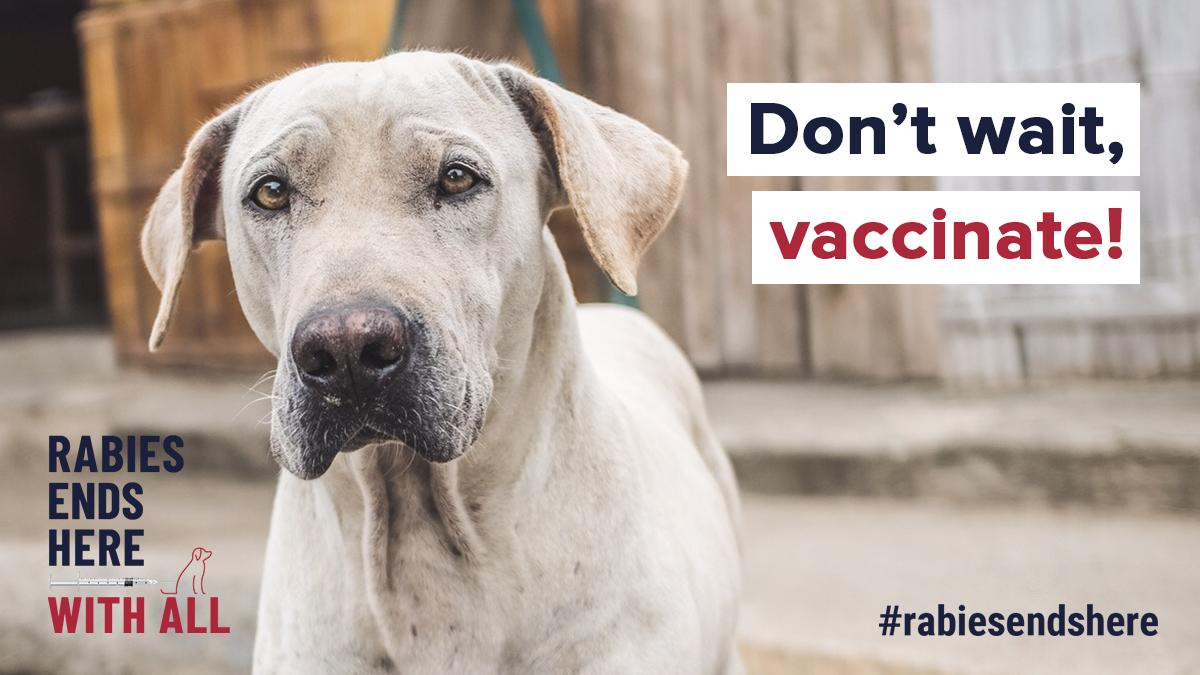The image showcases a graphic design poster centered around a poignant photograph of a forlorn-looking dog. The dog, predominantly white with black spots, has drooping ears, a black nose, and yellow eyes, projecting an overall sad demeanor. 

To the right of the dog, two white rectangles feature prominent textual messages. The upper rectangle bears the text "Don't Wait" in black (or possibly dark blue, according to another description), while the lower rectangle emphatically states "Vaccinate!" in striking red. On the left, similar design elements carry the message "Rabies Ends Here" in black, accompanied by a red "With All" beneath. Adjacent to these texts is a graphic depiction of a syringe and a dog outline.

In the bottom right corner of the poster, the hashtag "#rabiesendshere" is conspicuously placed. The blurred background hints at an urban setting with indistinct buildings and streets, adding context to the scene.